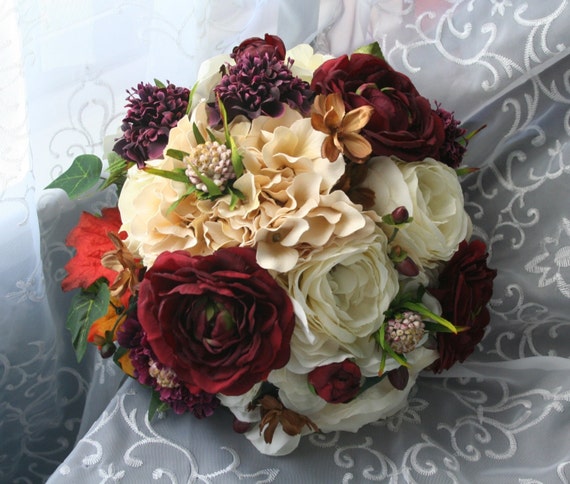This is a photograph of an elegant, round bouquet of roses, possibly designed for a bridal or bridesmaid setting, captured from a top-down perspective. The bouquet sits atop a draped, silky gray cloth adorned with swirling white filigree, reminiscent of veil material. The arrangement features a variety of roses: the majority are large, off-white and ivory blooms, interspersed with darker red roses, including a few deep burgundy ones. Complementing the roses are clusters of pink ball-shaped flowers and verdant green leaves, with additional pops of red and brown leaves towards the base. The intricate details and vibrant colors make this bouquet a stunning focal point against the sophisticated backdrop.